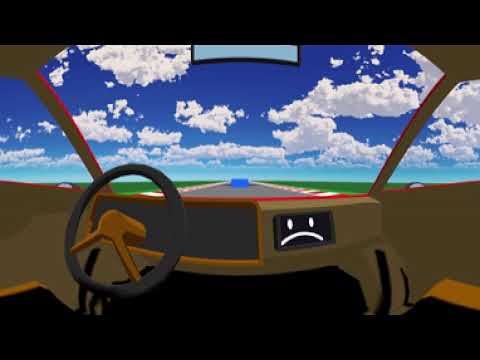The image is a rudimentary cartoon illustration depicting the interior of a car, viewed from the driver's seat. The perspective shows a black steering wheel with two downward spokes, which is set against a primarily orange-toned car interior. To the right of the steering wheel on the dashboard, there is a screen displaying a frowning face on a black background. Through the windshield, the road ahead is visible, resembling a track with black, white, and red barriers at the end and a blue barrier directly in front of the car. The surrounding scenery includes green grass on both sides of the road, under a sky that's a vivid blue, scattered with white clouds. The entire image is framed by black borders at the top and bottom, adding to the cartoonish vibe.